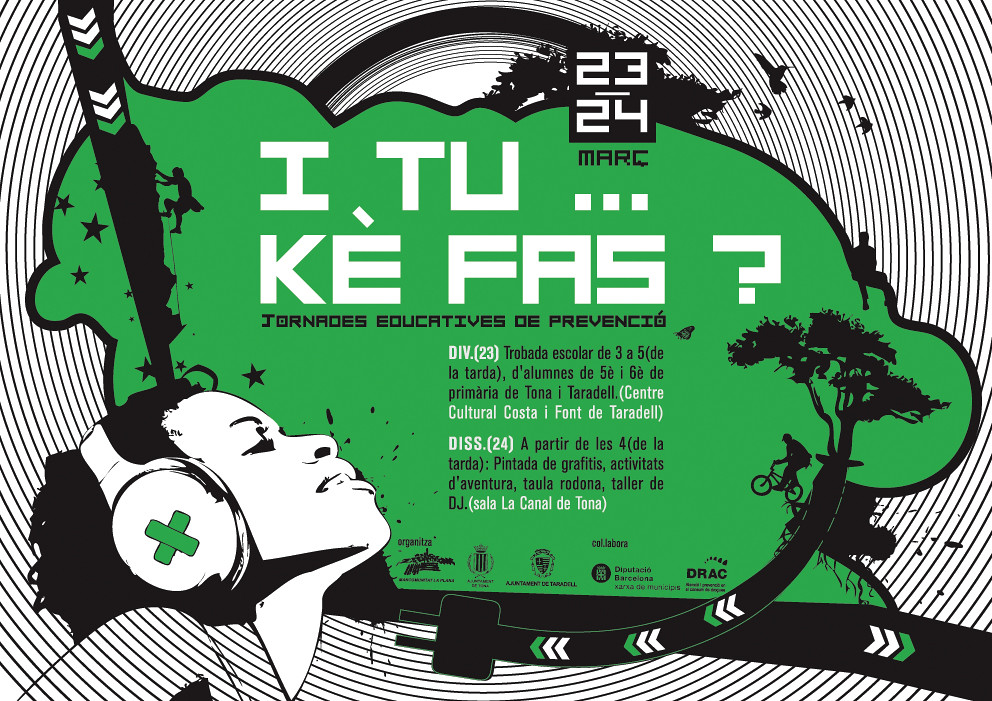This illustration is an advertisement poster, likely promoting an educational event named "Jornados Educativos de Prevención," happening on the 23rd and 24th of March. The poster features a multilingual mix of text, in both English and a Romance language, possibly Portuguese or Spanish. Central to the design is a medium green blob with yellow undertones, bordered by a black outline, which contains the key textual information. Prominently displayed in large white block letters is the phrase "2324 Març" followed by "I2KEFAS?" in white letters. Additionally, the poster lists specific event activities, including scholarly work from 3 to 5 PM by students of the 5th and 6th year of Primaria de Tona at Centro Cultural Costa Ponte de Tarradell.

The visual elements include a striking black and white profile of a multiracial woman on the left side. The woman, who appears to be of African descent, has short hair, wears headphones marked with a green X, and gazes upward. Spiraling black and white patterns form the background, with three sets of arrows pointing left and downwards interspersed around the green blob. The right side of the image features a tree with exposed roots, where a person on a bicycle is teetering on one of the roots, along with the depiction of a climber scaling a rock face. The bottom of the poster includes logos of various sponsors, indicating their support for the event.